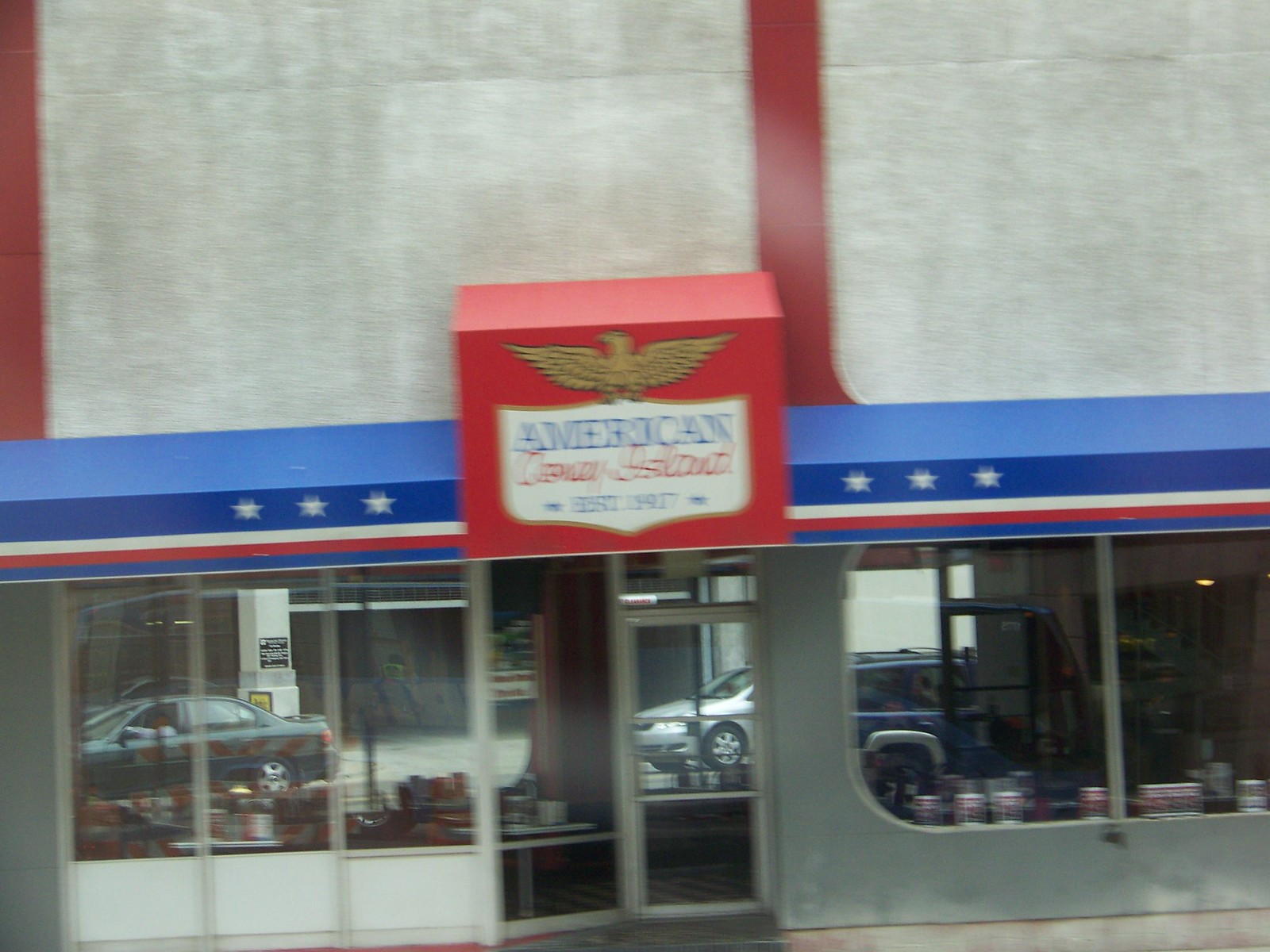This photograph captures an exterior view of a building, likely a storefront. The image is slightly blurry, suggesting it was taken while the camera was in motion. Reflections on the building's windows display several parked cars. Above the storefront, there's a prominent sign featuring the word "American" in clear, bold type. Below this, an indecipherable word in red cursive script hints at the establishment’s name or slogan, partially obscured due to the image's blurriness. The sign itself is mounted on a white, shield-shaped background, which is in turn set against a red rectangular box. Crowning this sign is a golden eagle logo, adding a touch of regality to the building’s facade. The upper section of the building is characterized by a stark, grey wall, giving the scene a somewhat industrial or utilitarian appearance.